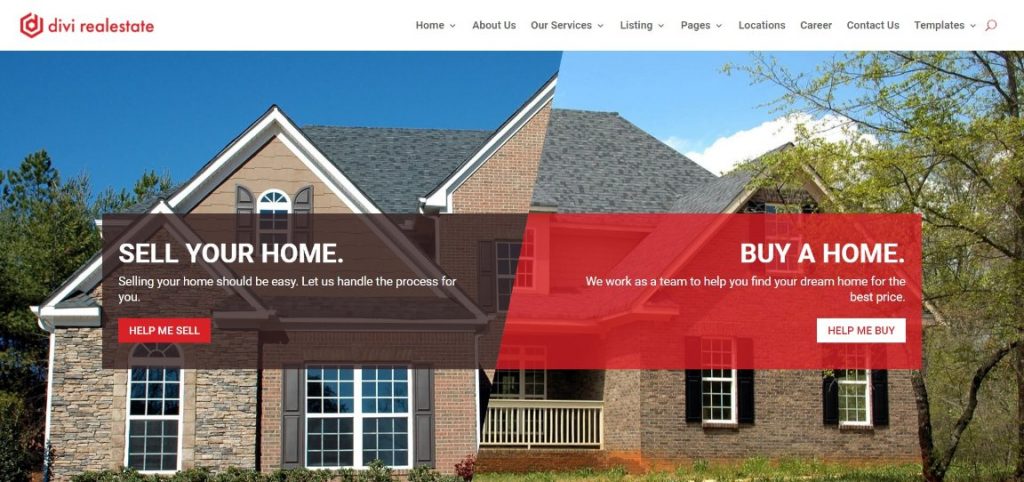The image features a detailed webpage for D-I-V-I Real Estate, presented in a structured and organized layout.

At the top, there's a prominent header with a white background on the left side, shaped somewhat like a hexagon. This section seamlessly transitions into a red background on the right. The text "D-I-V-I Real Estate" is displayed prominently. Below this, in black font, the navigation menu lists the following options: Home, About Us, Our Services, Listing, Pages, Locations, Career, Contact Us, and Template. A red magnifying glass icon indicates a search function.

The main section of the webpage showcases two large images of the same house, characterized by a gray roof and brown brick walls. The left side of the image displays a large brown rectangle with white text saying, "Sell Your Home." Below it, the message continues: "Selling your home should be easy. Let us handle the process for you." Adjacent to this message is a red rectangle with the white text, "Help Me Sell."

On the right side, there is another red rectangle with white text stating, "Buy a Home." Following this, the message reads: “We work as a team to help you find your dream home for the best price." Below this, a white rectangle with red text says, "Help Me Buy," all in capital letters.

In both images of the house, the sky is visible. The left image shows a clear blue sky with no clouds. The right image shows a lighter sky with some clouds partially obscured by green trees. Both images depict green grass at the bottom, adding a touch of natural beauty to the scene.